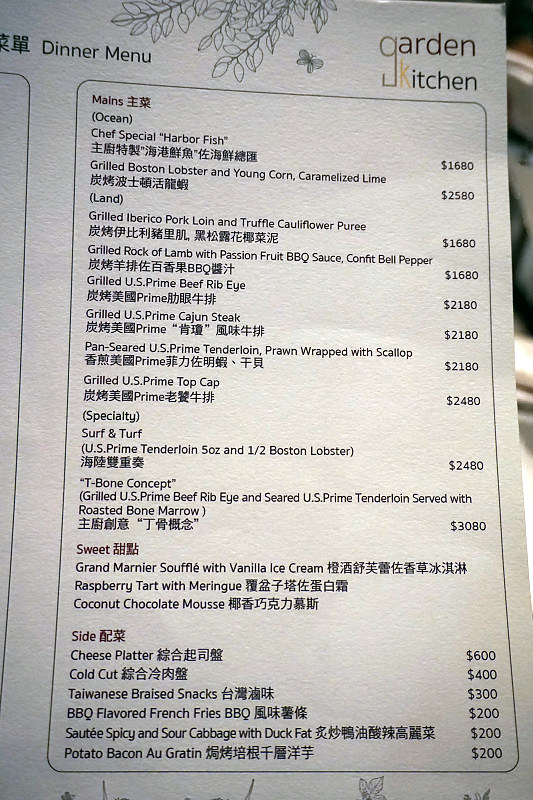A partially visible dinner menu is displayed on a textured white sheet of paper with a rounded black border. The top of the menu denotes "Dinner Menu" and features a hanging plant gently cascading from above. On the upper right-hand corner, the words "Garden Kitchen" are accompanied by Chinese characters and their English translations. The visible section of the menu lists various mains, sweets, and sides, each with prices in dollars, although notably high, such as a T-bone steak priced at $3,080. To the left, the edge of another part of the menu is faintly visible. In the background towards the right, a blurry ambiance can be seen, though its specifics are indiscernible, complementing the natural theme established by additional flowers and plants seen at the bottom of the menu.